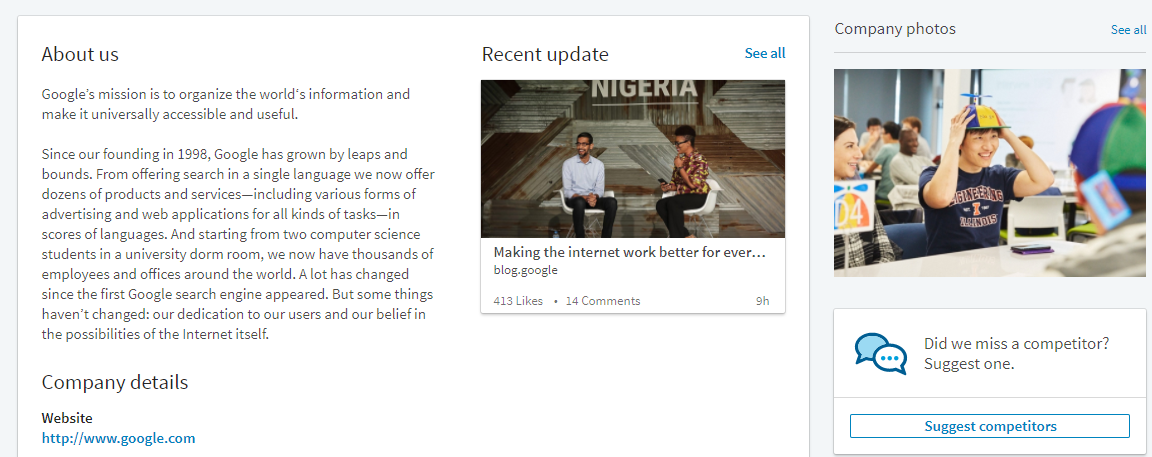Screenshot Overview:

The image presents a detailed and expansive screenshot of Google's "About Us" section from their website. The section articulates Google's mission statement: "To organize the world's information and make it universally accessible and useful."

Detailed Description:

At the top of the screenshot, the mission statement is prominently displayed, emphasizing Google’s commitment to accessibility and usability of global information. Below this, a paragraph chronicles the history of the company, noting its substantial growth since its inception in 1998. Despite the vast changes since Google's early days as a nascent search engine, the text underscores the company's unwavering dedication to its users and its core beliefs in the possibilities of the internet.

The screenshot also includes a link directing to an article featuring Sundar Pichai, the CEO of Google, although his name is not mentioned explicitly in the voice note. Further down, several company photos are shown; one notable picture captures a young Asian engineer, who, despite having the appearance of a stock photo model, might be a genuine employee. He is depicted wearing a playful propeller hat and a dark navy t-shirt, embodying the fun and innovative culture at Google. This lighthearted imagery reinforces the company’s creative and vibrant work environment.

In summary, the screenshot offers a comprehensive glance at Google's ethos, historical journey, and the engaging work culture that continues to steer the company forward.